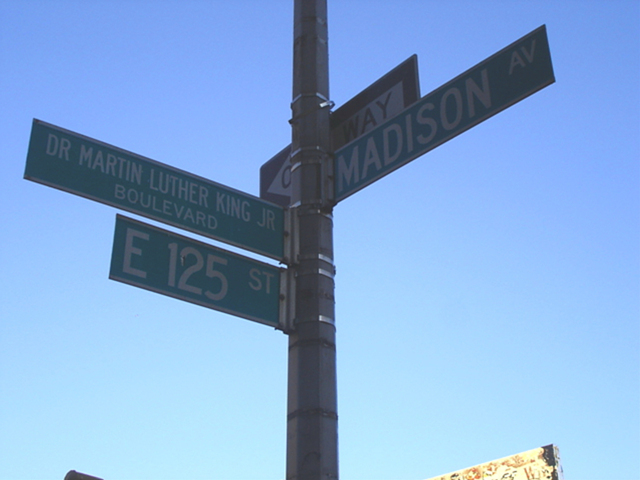In the image, a tall metal pole supports several street signs against the backdrop of a clear blue sky. At the top left, a green sign with a white border and white capital letters reads "Dr. Martin Luther King Jr. Boulevard." Directly beneath it, another green sign with white lettering indicates "E-125 Street," where "E" likely stands for "East." On the pole's left side, yet another green sign with white letters points to "Madison Ave." On the right side of the pole, a black sign with white text, partially obscured by the pole itself, seemingly reads "One Way" and directs traffic in the opposite direction.